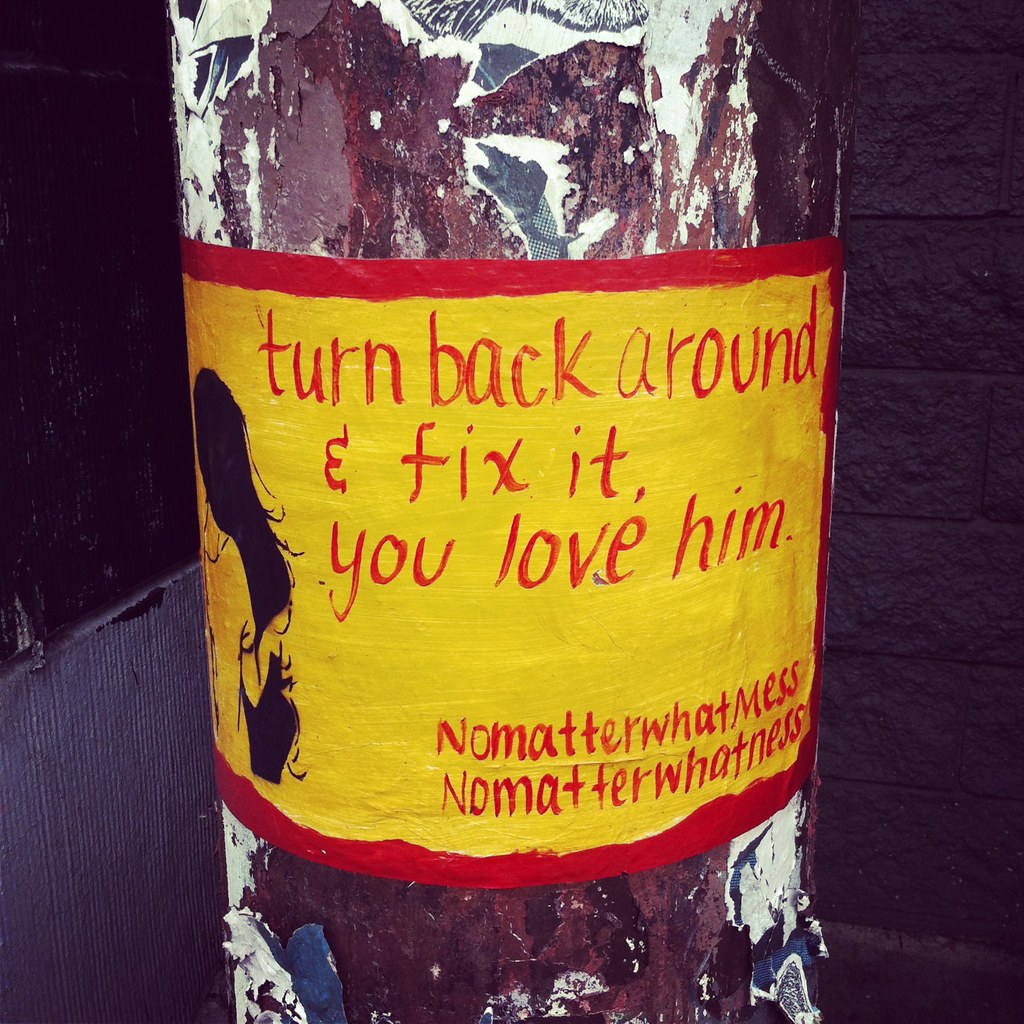In the center of the image, a cylindrical object, perhaps a tree trunk or a pole, commands attention. It's sheathed in reflective aluminum foil, giving it a standout appearance against its surroundings. The object's surface is adorned with a vibrant yellow flyer bordered in red. The flyer bears a poignant message in red text: "Turn back around and fix it, you love him. No matter what mess, no matter what mess."

The background features a context of decay, with a dilapidated brick wall to the right and a crumbling structure to the left, emphasizing an atmosphere of neglect or abandonment. The colors within the scene range from grays, blacks, and browns of the deteriorating walls, to the stark whites and tans of the surrounding area, juxtaposed against the striking red and yellow of the flyer. Positioned directly in the centre, this enigmatic, possibly rusty and weathered, bottle-shaped object with its heartfelt message draws the viewer's focus in a setting that appears both artistic and evocative.